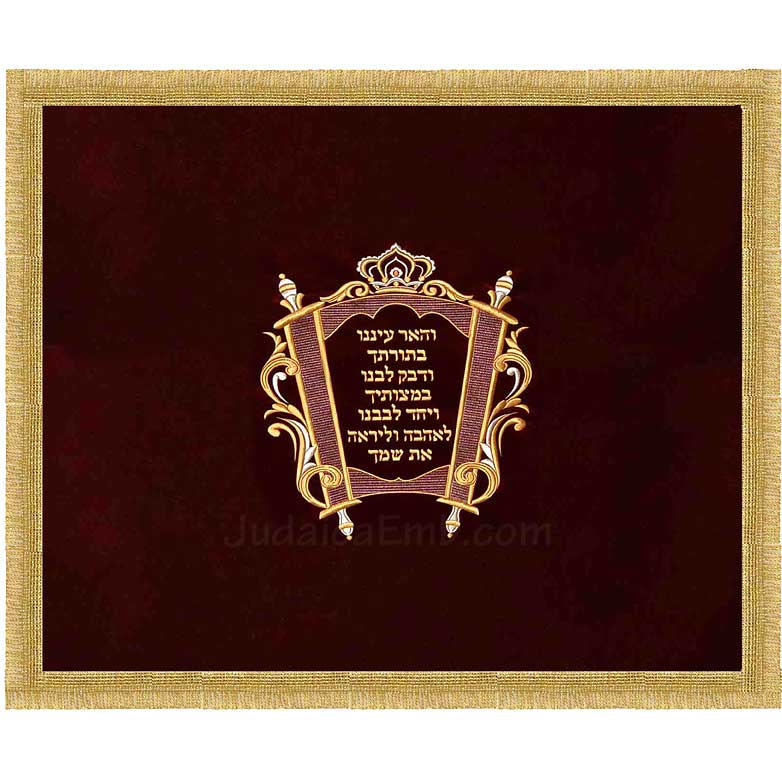This image showcases a richly detailed fabric wall art piece, perhaps a religious tapestry intended for display in a synagogue. The tapestry is square, featuring a uniform, neat border of golden, woven fabric tassels that frame a dark, velvety central background. This background, a deep and subtly textured blend of black and burgundy hues, houses a central embroidered image of a Torah scroll with rounded top edges. The scroll is adorned with intricate gold filigree decorations and a crowned top. Hebrew lettering in gold embellishes the central area of the scroll. The craftsmanship of the tapestry, including the tassels, gold embroidery, and the detailed Torah depiction with its accompanying decorations, underscores its religious significance and artisan quality.